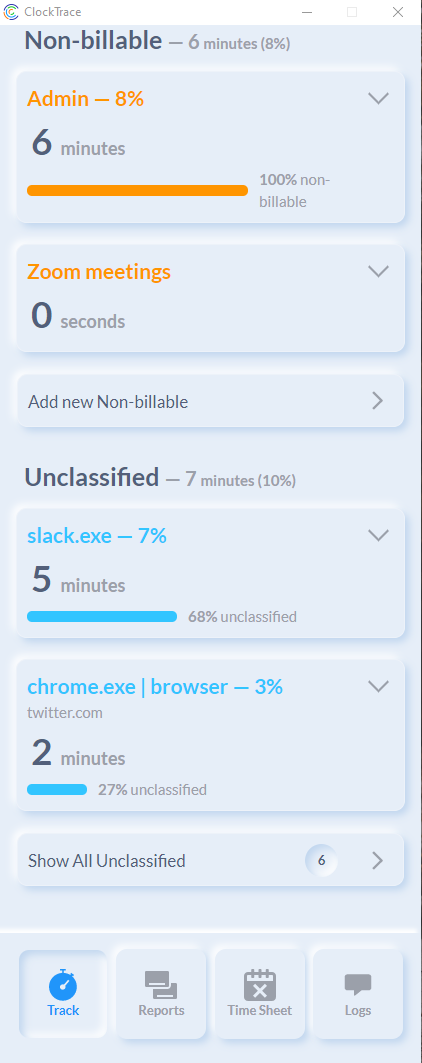This image is a screenshot of a digital time-tracking application interface. The screenshot captures the content of the screen, showcasing a website in the browser on a device. At the top left corner, there is a header that reads "Clock Trace," accompanied by an icon. On the right top corner, the area is in white and features a minus symbol enclosed in a box followed by an "X" for closing the window.

Beneath the header, there's a section labeled "non-billable," presented in gray. Here, a minus sign precedes the text "six minutes" (formatted as "-6 minutes"), with "8%" indicated in parentheses. Below this, in a boxed section labeled "admin," an orange-highlighted text shows "-8%," and beside it, a drop-down arrow is available. The same box displays "six minutes" again, with a corresponding orange progress line filled up to 100%.

A similar format is observed in the "Zoom meetings" section, which is noted to be at zero seconds and includes a drop-down arrow. Below this area is an actionable text link that reads "Add new non-billable" with an arrow pointing to the right.

Farther down, the "unclassified" section mentions "seven minutes." It includes another drop-down box specifying "slack.exe - 7%," totaling five minutes with a blue progress line reaching 68%. Next to this is indicated "Chrome XE browser" with two minutes tracked and another drop-down arrow.

At the bottom of the screenshot, there are several buttons, including "Show all unclassified," "Track," "Reports," "Timesheets," and "Logs," providing navigational options for the user within the application.